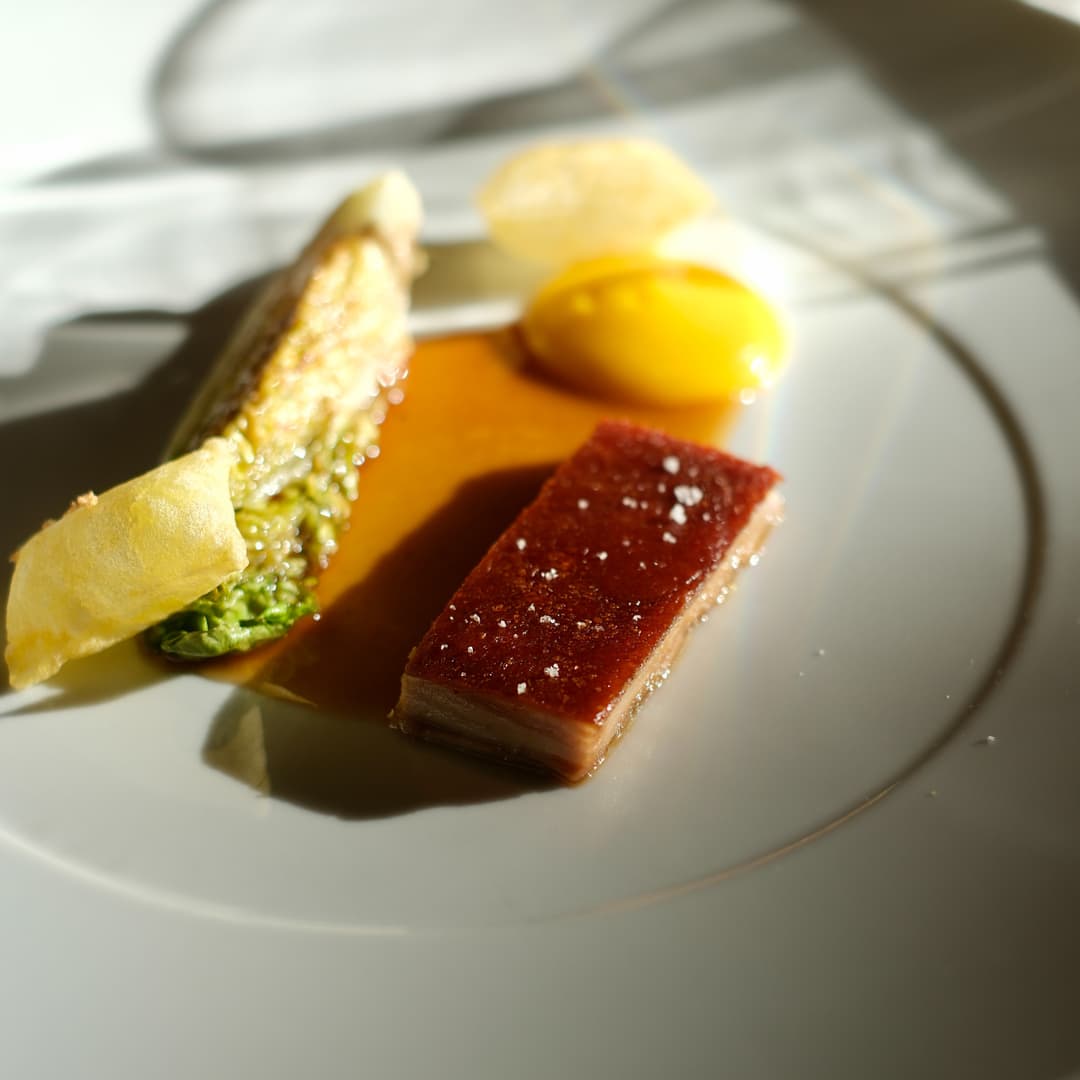This is a color photograph showcasing an elegantly plated fine dining dish on a simple yet sophisticated white plate with a gold band. The focus of the image is on a small section of the plate, with the closest items in sharp clarity while the distant items fade into a soft blur. At the forefront, there is a meticulously layered, rectangular bar the size of a business card, topped with a red fruit spread and sprinkled with crystalline accents, which could be salt or sugar. Adjacent to this is a delicate wrap resembling half of a crepe, filled with finely cut vegetables and resting within a pool of light brown sauce. Nearby, there is a pillow-like puff pastry, filled with a green filling, and positioned further back is something that looks like a vibrant yellow egg yolk. The overall composition suggests a sophisticated, European-inspired dish, likely from a fine dining establishment, featuring small, artfully arranged portions that highlight the culinary artistry.